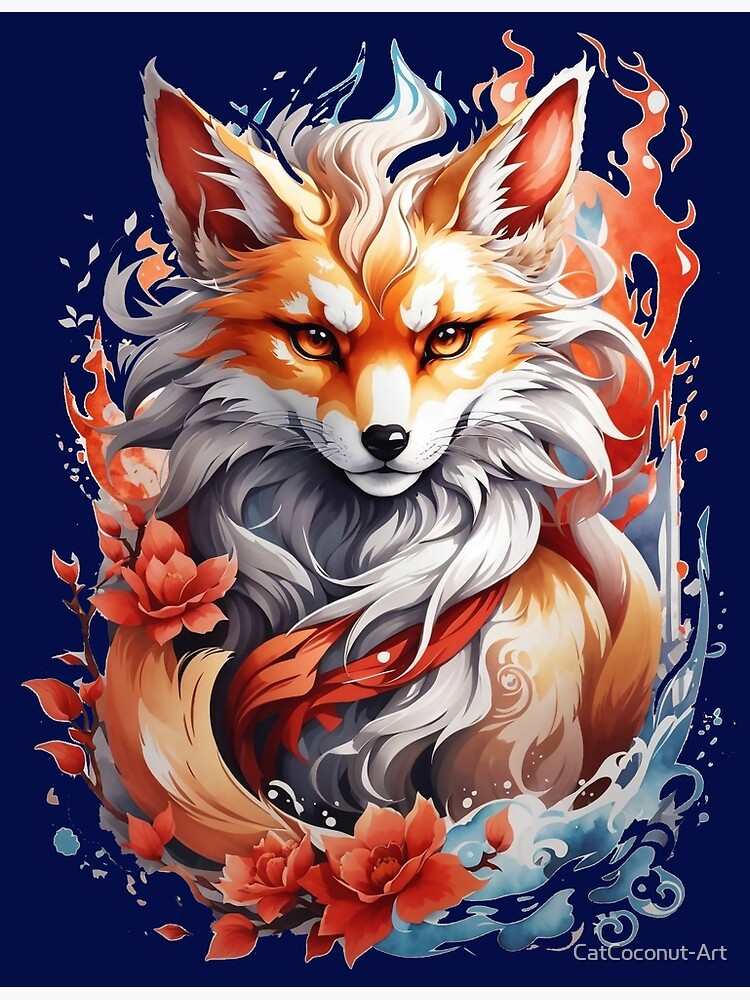This vibrant and striking piece of art, titled "Cat Coconut Art" in light blue text on a dark blue background, features a brilliantly animated, almost cartoonish depiction of a fox. The fox's face is the centerpiece, with its vivid orange fur, large amber eyes, and a black nose. The fox's ears, looking like flames, add to the dynamic appearance. White fur cascades from its nose area and down its neck, extending between its ears. Surrounding the fox’s head is a fiery, almost ethereal substance that enhances the artwork's dynamic quality.

The lower portion of the image is adorned with orange flowers, placed predominantly at the bottom and to the left. Additionally, the bottom right corner contains a white and light blue area that resembles smoke or fire, adding depth and texture to the scene. The fox’s tail is depicted as full and bushy, wrapping around its lower body, contributing to the three-dimensional aspect of the artwork. This stunning and detailed portrait captivates with its blend of natural and fantastical elements, leaving a lasting impression and inviting viewers to interpret its rich details.